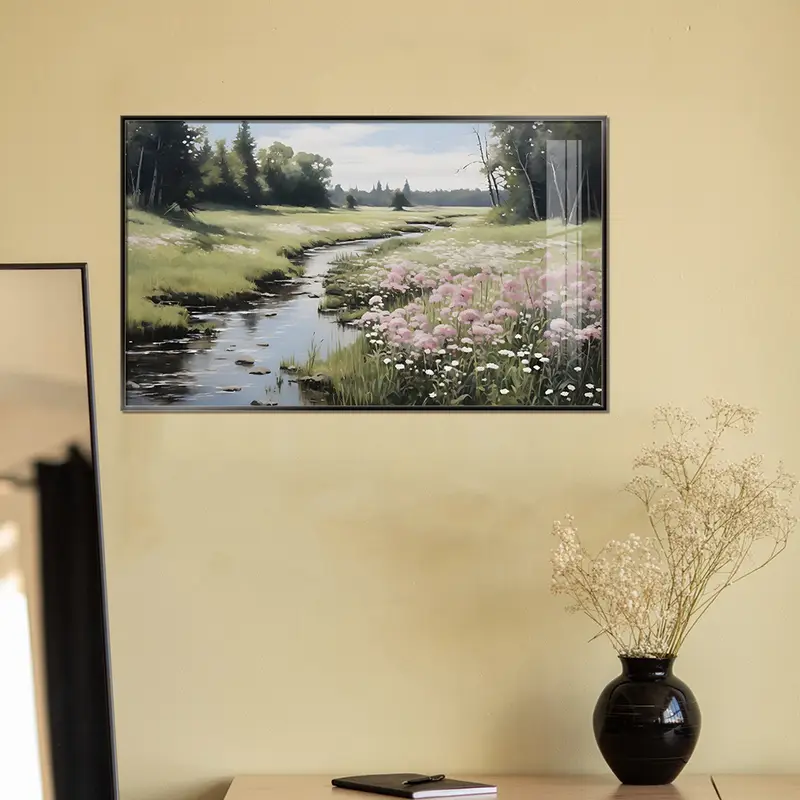A square color photograph captures the tranquil interior of a room dominated by a light yellow wall. Centrally placed near the top part of the image, a horizontally oriented framed print portrays a serene scene of a stream or marshlands, adorned with a field of pink and white flowers. The print is protected by a plastic or glass cover and is encased in a gray or possibly black frame.

From the lower left corner, a secondary frame—likely a mirror due to its reflective surface—extends upwards toward the center of the photograph, though its reflection is indistinct and blurry. Anchoring the bottom of the image is a low wooden table, upon which rests a round glass vase filled with dried flowers. Adjacent to the vase, positioned to the left center of the table, lies a composition notebook with a pen placed on top of it.

Subtle shadows stretch across the table, cast by the vase, while highlights softly illuminate the glass, enhancing the room's serene ambiance.